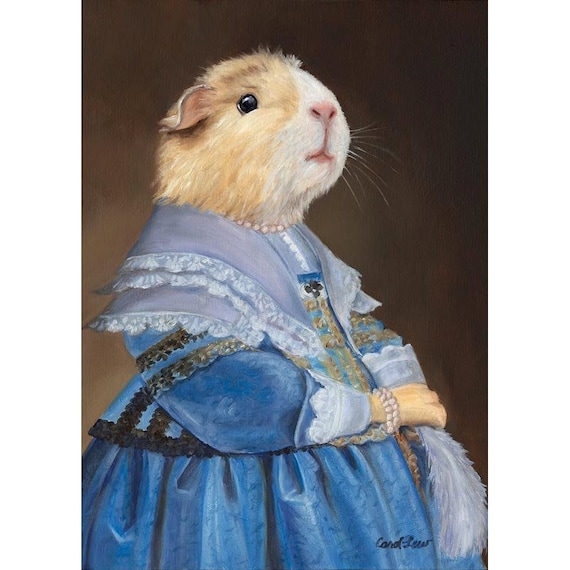The image depicts a meticulously detailed and talentfully crafted representation of a guinea pig, illustrated or possibly digitally manipulated to appear as though it belongs to the Elizabethan era. The guinea pig, with its black eyes, distinctive white and light brown face, and pink nose and mouth, exudes a lifelike charm. Its ears, a mix of light brown and somewhat floppy, add to the authentic guinea pig visage, complemented by white whiskers. The background of the image is brown, setting a warm, neutral scene.

Adorned in an elaborate, light blue dress with gold ribbon trim and slightly ruffled light whitish-blue sleeves, the guinea pig exudes an air of nobility. The dress features white chiffon details around the neck and shoulders, enhancing its regal appearance, and is accentuated by elegant gold embroidery down its middle. The guinea pig is further accessorized with a delicate string of pearls around its neck, emphasizing its genteel portrayal. In its paw, it delicately holds a white feather or possibly a quill pen, hinting at a historical or creative context. The image bears an unreadable signature scrawled in black at the bottom, signifying the artist's mark. The entire scene is framed vertically in a rectangular layout, giving this charming figure a portrait-like quality.